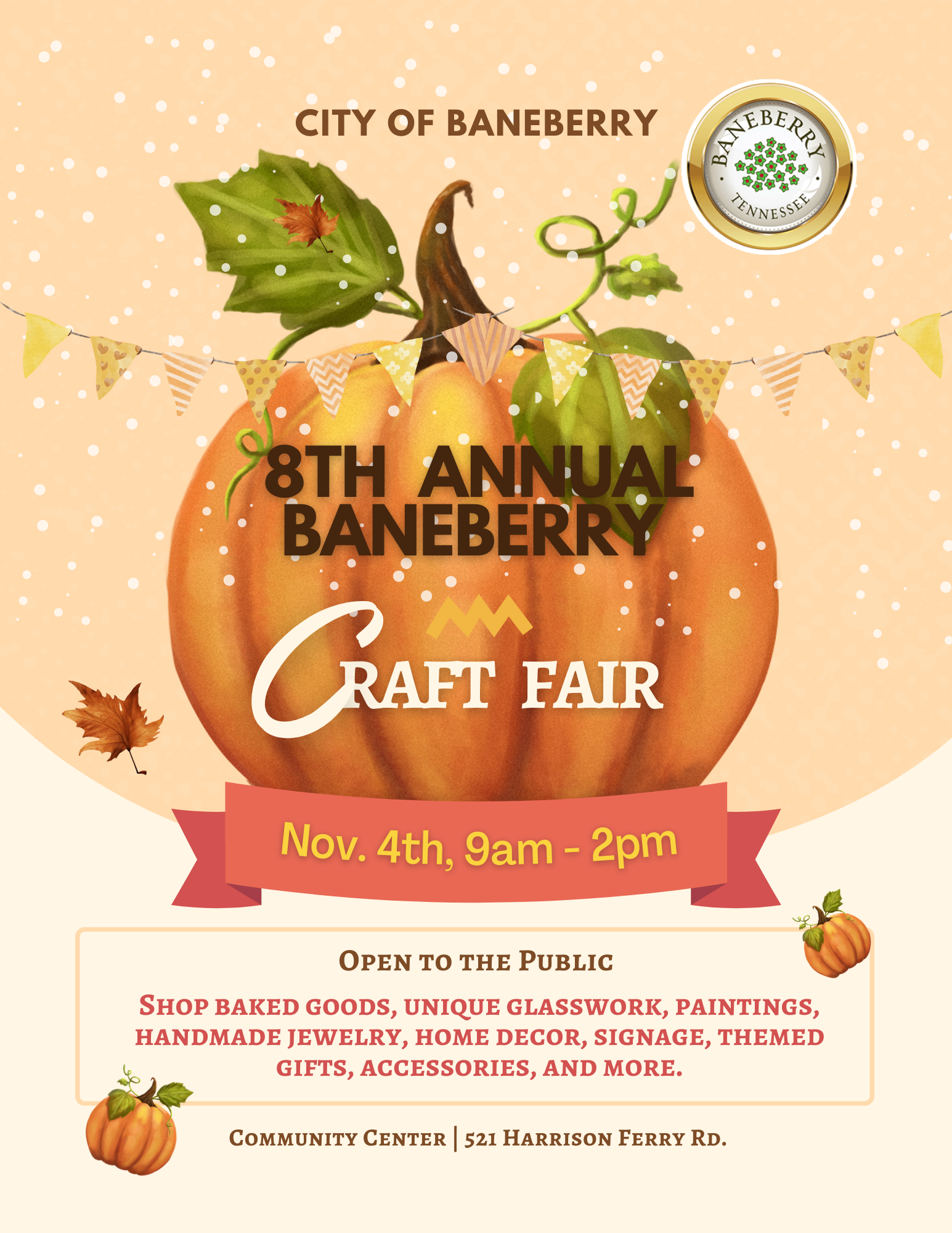The image features a festive flyer with a warm, peachy-orange background speckled with white dots. Centered at the top, in elegant brown font, it reads "City of Bainbury." Beneath this, a standout pumpkin graphic with a green leaf and stem takes center stage. Inside the pumpkin, "8th Annual Bainbury Craft Fair" is prominently displayed in larger brown text. Just below the pumpkin, a red and orange ribbon spans horizontally, with the event details "November 4th, 9 AM to 2 PM" written in bright yellow.

In the upper-right corner, there's a small logo, and alongside it, a smaller leaf motif, perhaps an oak leaf. Text within a white border box, accented by pink lines, states: "Open to the public. Shop baked goods, unique glasswork, paintings, handmade jewelry, home decor, signage, themed gifts, accessories, and more." Additional elements include two tiny pumpkins positioned in the upper right and lower left corners of the box.

At the bottom, the address of the event is noted: "Community Center, 521 Harrison Ferry Road, Bainbury, Tennessee."